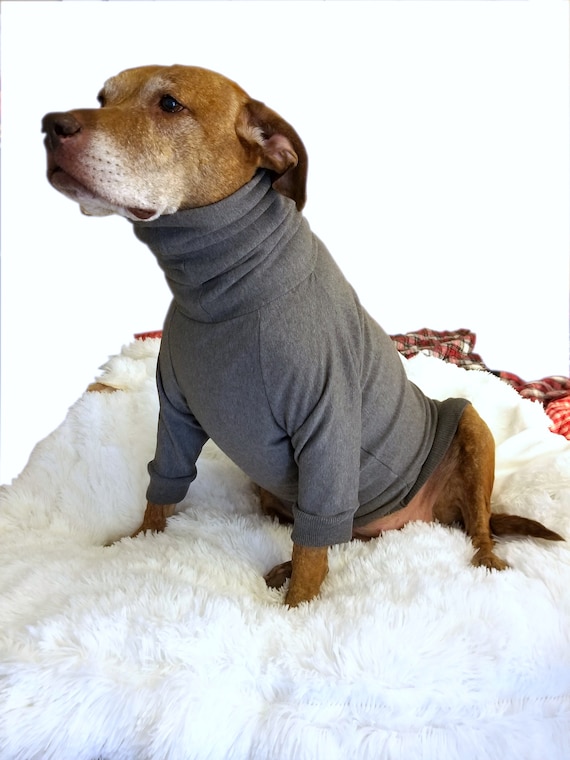This detailed photograph captures an elderly brown dog sitting lopsidedly on a bright white, shaggy, fake fur rug. The dog has a mix of grey and brown fur, indicative of its senior age, and sports a long-sleeve, grey turtleneck sweater that ruffles and covers its whole neck down to its forepaws and waist. The dog has a white muzzle and ears laid back, giving it a contemplative expression as it gazes slightly to its right, approximately at a 45-degree angle. The background, although predominantly white, shows hints of red patterns from a blanket or clothing item. There is also some additional clothing visible in the background, likely part of the bedding.